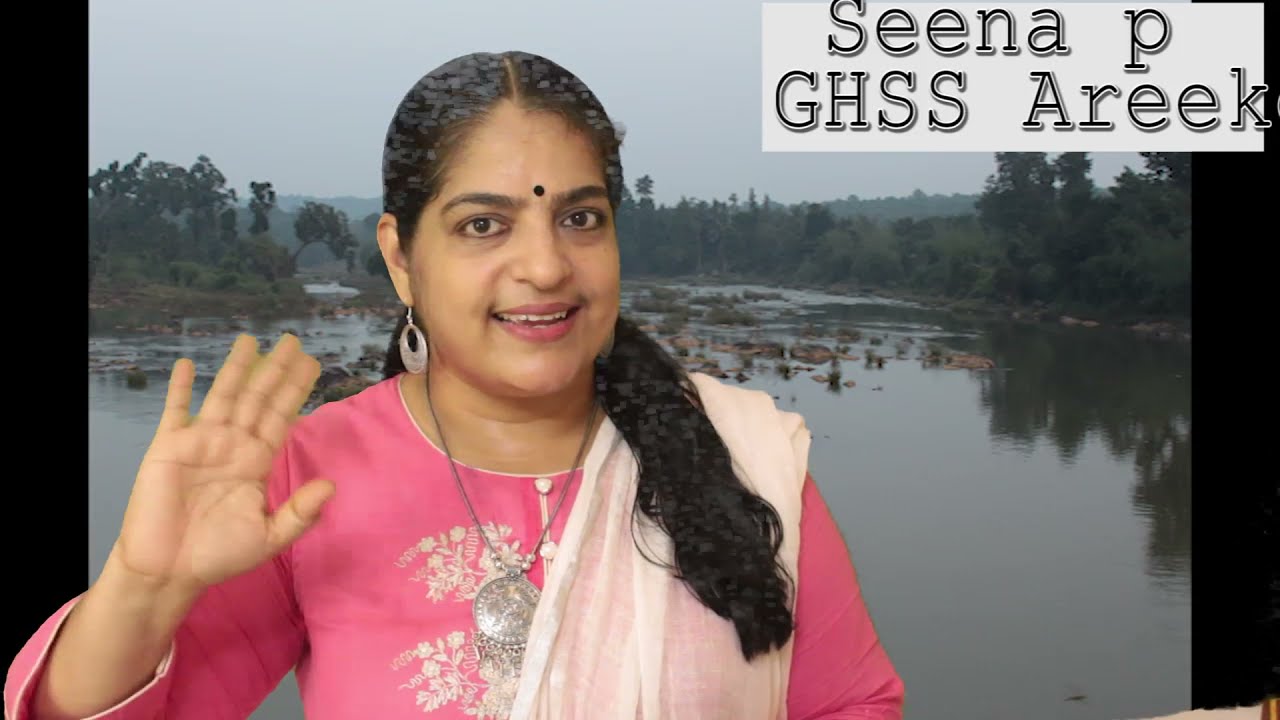The image depicts an Indian woman standing in front of a misty lake with distant green trees and a grayish-blue sky, reflected on the water's surface on the right side of the image. The woman, dressed in a pink dress, waves at the camera with her right hand, displaying a warm smile with her teeth slightly showing. She has long black hair pulled back with part of her ponytail resting over her left shoulder. Her attire includes a pink sash crossing diagonally from her left shoulder, a silver medallion necklace, and silver hoop earrings. A bindi adorns her forehead, and she wears lipstick and eye makeup. In the top right corner of the image, a white rectangular box with black text reads "Sina P G H S S Arik."